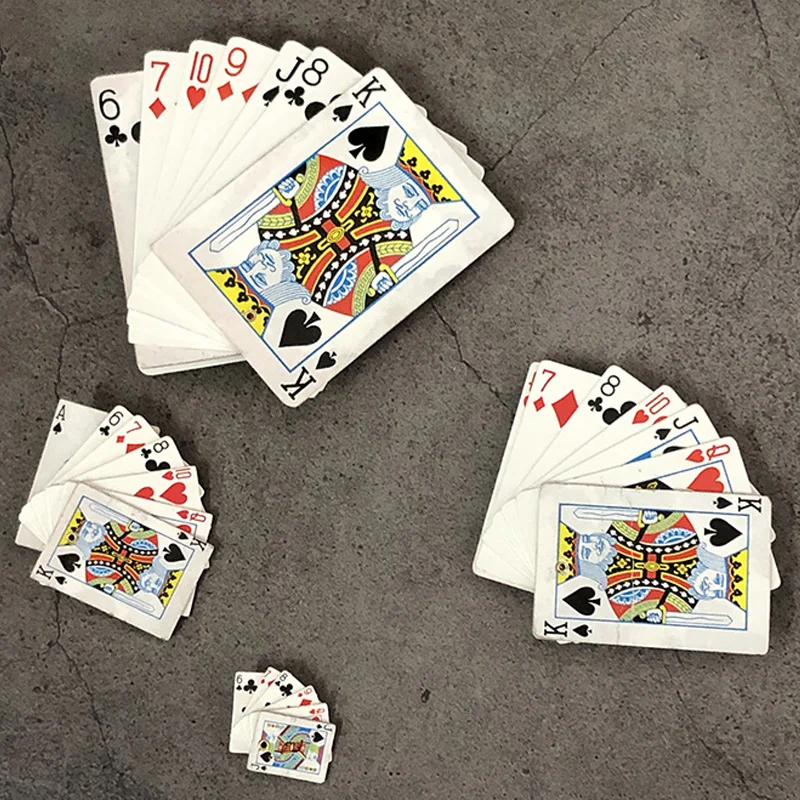The image depicts four stacks of playing cards arranged on a concrete pavement with noticeable hairline cracks. Each stack contains multiple cards fanned out in a semi-circular fashion. Three of the stacks notably feature a King of Hearts as the top card, each followed by six other cards. These stacked hands vary in sizes, with the largest stack located at the upper left. This dominant stack comprises Kings of Hearts and various cards of different denominations and suits, including clubs, diamonds, hearts, and spades. To its right lies a smaller stack, also topped with a King of Hearts, and similarly consisting of a mix of red and black cards. The third stack, positioned to the immediate left of the second stack, is smaller yet, with the same King of Hearts configuration. The fourth and smallest stack deviates by having a Jack of Hearts as its top card, and also contains cards of different colors and suits. The overall scene is set against a gray stone or concrete surface, adding a stark, textured background to the colorful array of playing cards.